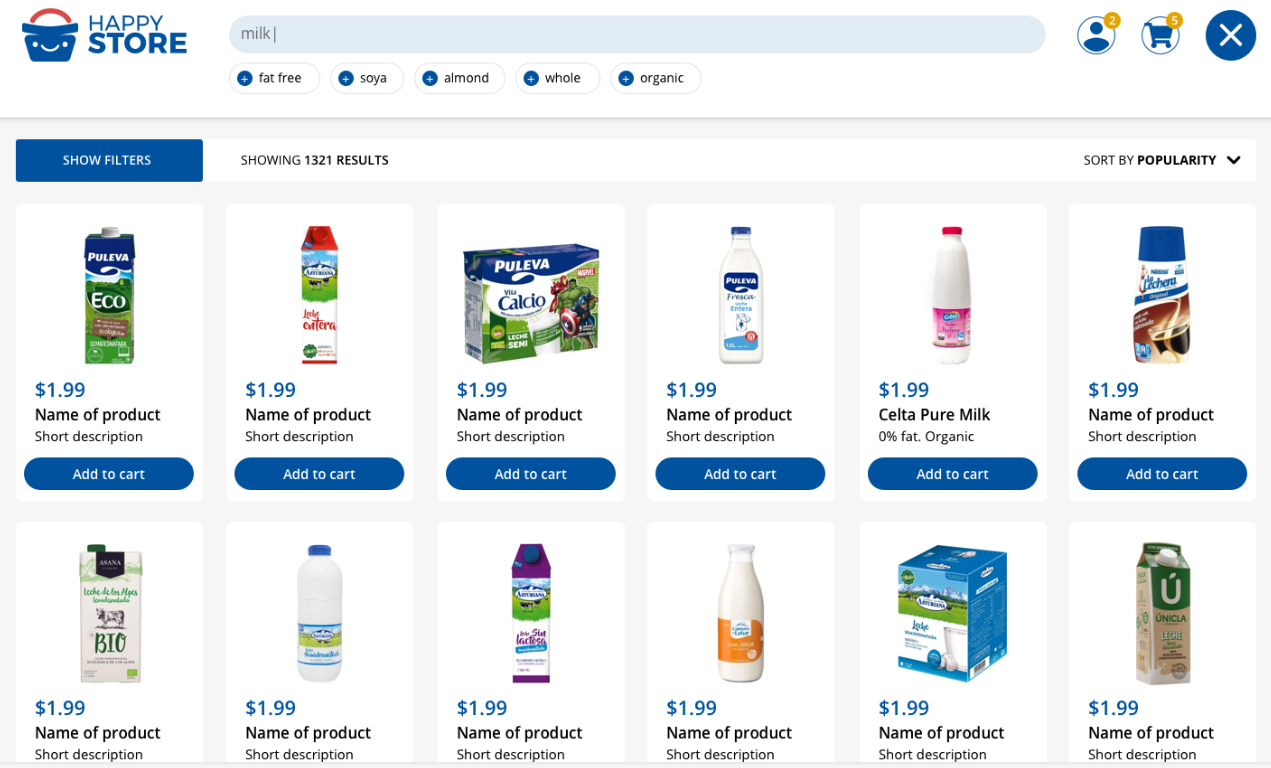"Shopping interface on The Happy Store website, featuring a variety of milk products"

The image showcases the online shopping interface of The Happy Store. The store's logo, a smiley face on a shopping basket with an orange handle, is prominently displayed. In the search bar, the word "milk" is typed. To the right, there is a user profile icon and a shopping cart icon next to a blue circle with an 'X' inside it. The page displays options such as "fat-free," "soy," "almond," "whole," and "organic" under a filter section, with an active blue box labeled "Show Filters."

Below these filters, the interface is organized into white product squares laid out on a gray background, with the page indicating a total of 1,321 search results. Items are sorted by popularity. Each product item is vividly colored and involved different types of milk presented in various packaging formats — bottles, boxes, cartons, and plastic containers. Every product square includes the name of the milk product, a brief description, and the consistent price of $1.99. A blue "Add to Cart" button is located beneath each product image, allowing for easy purchase options for the shopper.